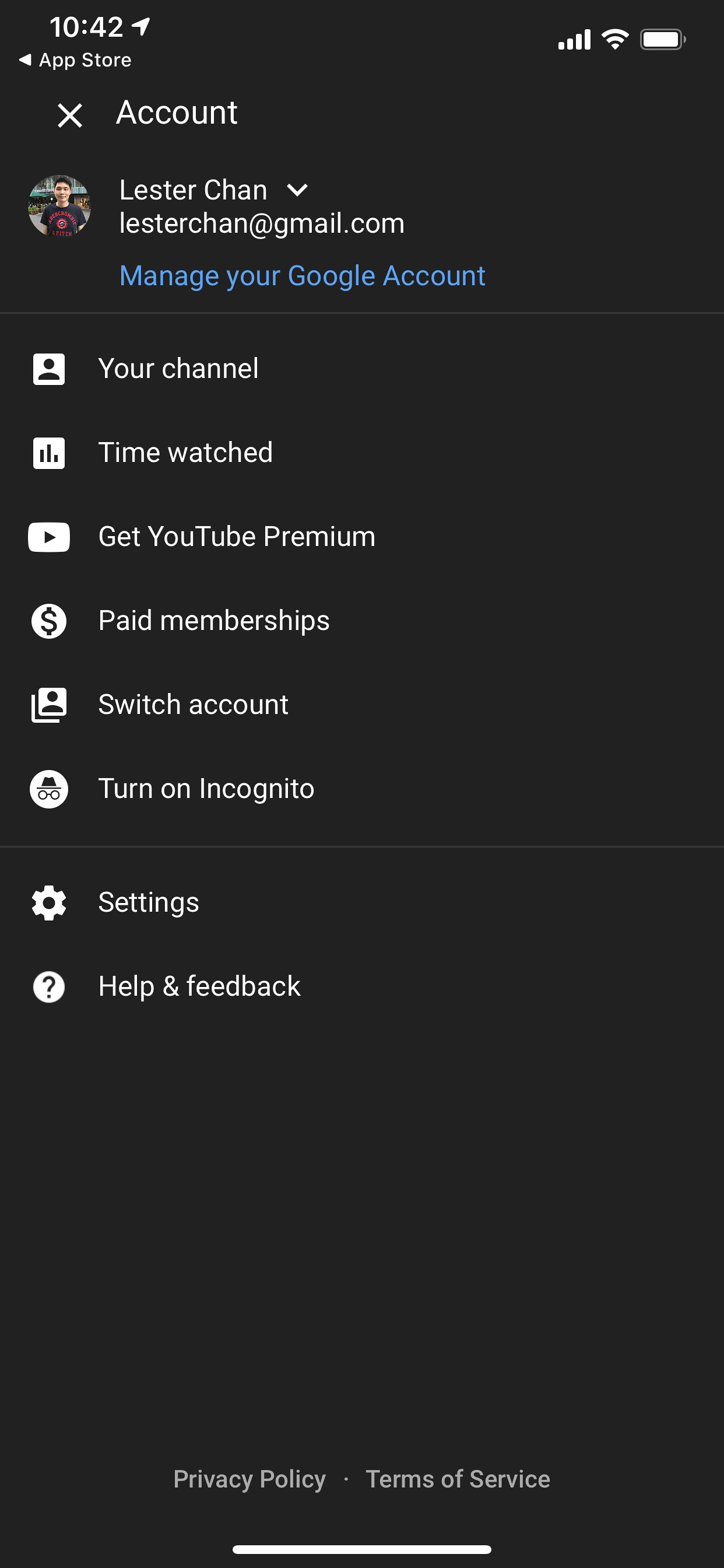The image is a detailed screenshot of a YouTube account displayed on an iPhone. In the upper left corner, the time is shown as 10:42 AM, and an icon indicates that the phone's location services are active. The interface shows options that include: “Your channel,” “Time watched,” “Get YouTube Premium,” “Paid memberships,” “Switch account,” “Turn on Incognito,” “Settings,” and “Help & feedback.” The account belongs to Lester Chan, as evidenced by the email address lesterchan@gmail.com. At the very bottom, clickable links for “Privacy Policy” and “Terms of Service” are visible. The iPhone's interface includes a white bar at the bottom center, which is typically used for swiping up to exit the app. The status icons show that the phone has four bars of cellular service, full Wi-Fi signal, and an almost fully charged battery. The application is displayed in dark mode, providing a sleek, modern look to the interface.